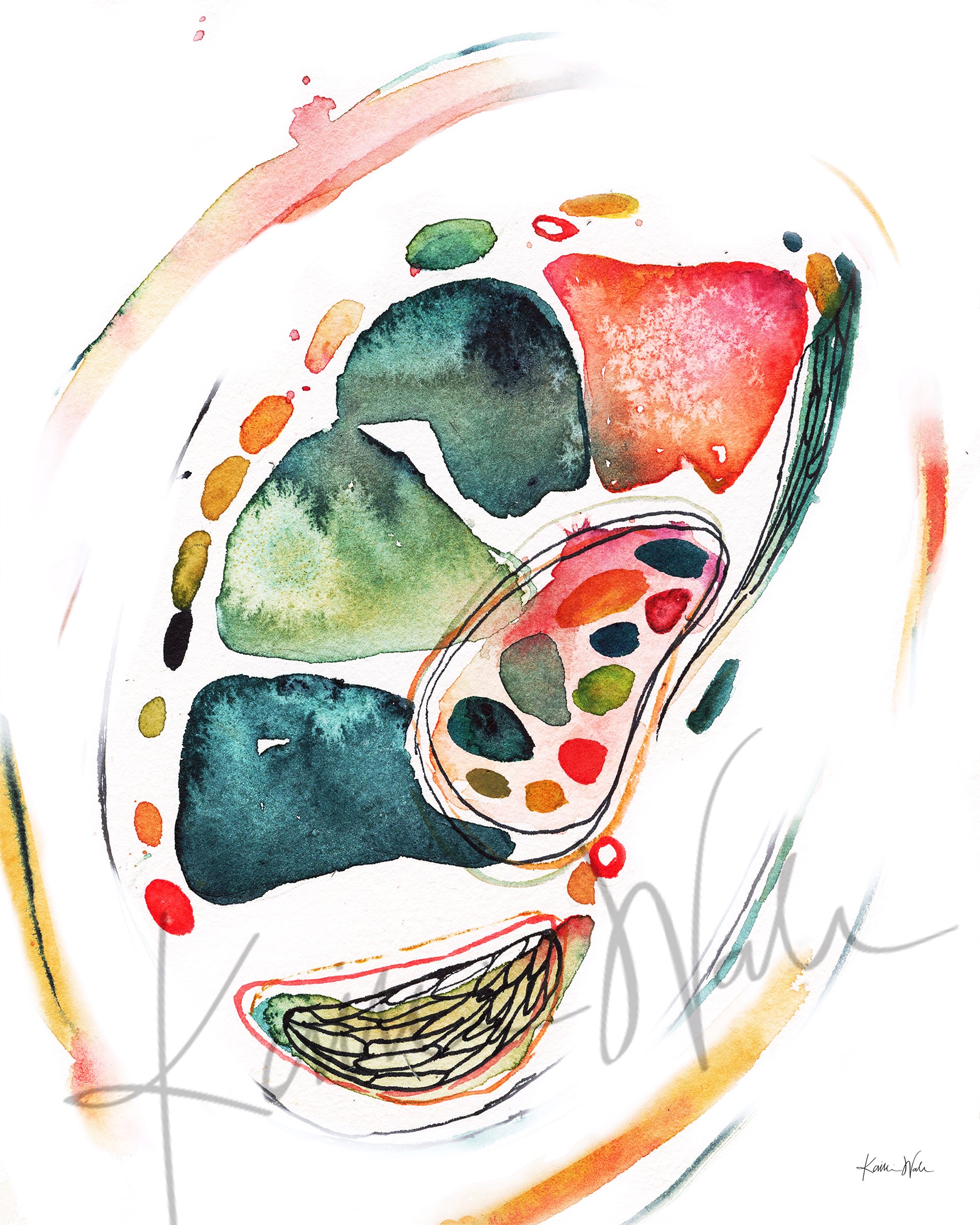This is an abstract painting characterized by its multi-color artistic splotches and irregular patterns. The artwork is vertically rectangular with no border and has a white background, as seen on the screen. Dominating the composition is an oval-shaped outline extending from the bottom left to the upper right, within which an eclectic array of colors is dispersed. The top left corner features a prominent pink swoop, while the lower left corner showcases a combination of green and yellow hues. In the center bottom, there is a distinct red bean-shaped form infused with intricate black lines.

Inside the oval are scattered splotches of colors including blue, green, and red with patches of white interspersed. These colors appear to form big areas that start in the middle, curve upward, and shift right, creating a dynamic and visually stimulating progression. Additional colors like orange and yellow appear towards the right, mingling with the white gaps throughout the image.

Notably, a small signature reading "VALX" is located towards the bottom of the painting, with another less readable inscription in the very bottom-right corner. The complexities and overlapping shapes give the impression of an artist’s easel, brimming with used paint and brushes, heightening the sense of abstraction and creativity.